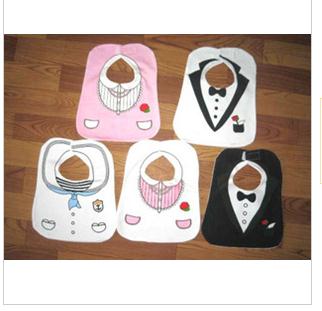The image features a set of five baby bibs, each uniquely designed to resemble adult clothing. The bibs are displayed on a wooden floor, adding a rustic touch to the setting. 

Starting from the top left, the first bib is pink with a graphic of a cap at the top, featuring a red rose and two white pockets. Adjacent to it, on the top right, is a black tuxedo bib. It showcases a formal design with a black bow tie, three white buttons, and a red flower in the pocket. Moving to the bottom left, there’s a bib designed to mimic a sailor outfit. This white bib includes black and white stripes near the collar, a blue tie, and a small animal figurine adorning the chest, accompanied by three white buttons.

Next to the sailor bib, the fourth item is a white tuxedo bib with black collars, a black bow tie, three black buttons, and a red flower in a black pocket. The final bib, located on the bottom right, has a white base with a cap graphic detailed with a pink and white striped visor, a red rose, and two pink pockets.

All five bibs combine playful and sophisticated elements, making them standout pieces for infants while mimicking grown-up attire.